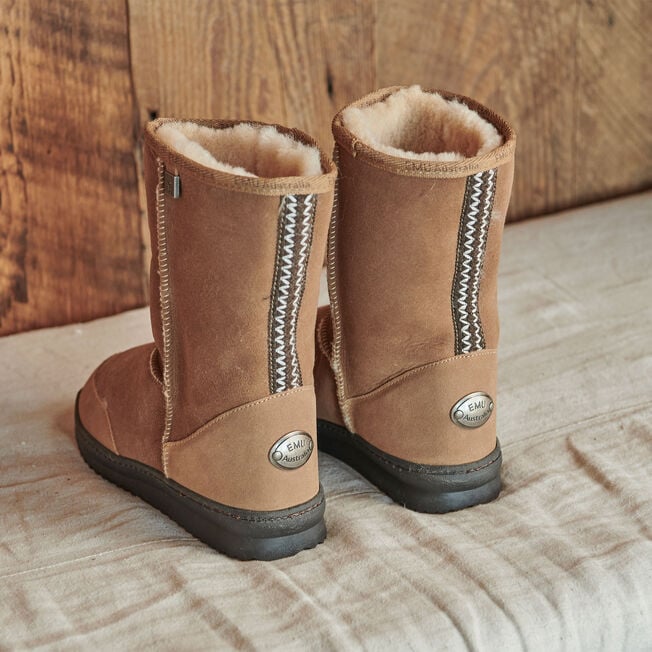This photograph features a pair of fashionable, casual winter boots viewed from the back perspective, with the heels positioned towards the bottom right corner and the toes pointing to the upper left. The boots are calf-high and display a buckskin color at the top and along the shaft. They rest on a textured tan cushion with various ridges.

A dark brown sole extends slightly up the boot, complementing the detailed design on the back seam. This back seam boasts a darker brown strip adorned with white zigzag stitching, adding a subtle yet stylish touch. Enhancing their practicality, the boots feature zippers on the outer sides. For added warmth and comfort, the interior is lined with tan shearling. At the heel of each boot, a metal emblem prominently displays the brand: "EMU Australia," with "EMU" in capital letters and "Australia" in lowercase except for the "A."